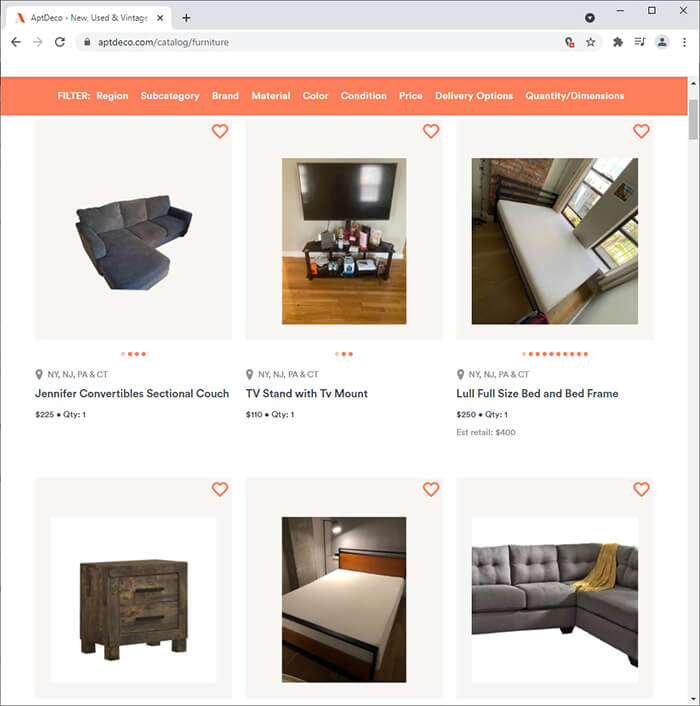This is a detailed screenshot from the website aptdeco.com, specifically from the catalog section showcasing furniture items. At the top, the URL displayed in the search bar is "aptdeco.com/catalog/furniture". Prominently, the heading reads "AptDeco – New, Used, and Vintage" followed by an orange banner featuring various menu options such as "Filter Region", "Subcategory", "Brand", "Material", "Color", "Condition", "Price", "Delivery Options", and "Quantity/Dimensions".

1. The primary section features:
   - A photograph of a black sectional couch with the caption reading, "NY, NJ, PA and CT, Jennifer Convertible Sectional Couch, $225, quantity: one".
   - An image of a TV stand topped with a flat-screen TV and scattered miscellaneous items. It is described as, "NY, NJ, PA and CT, TV stand with TV mount, $110, quantity: one".
   - A photograph of a mattress placed on a black bed frame, labeled "NY, NJ, PA and CT, Lull Full-Size Bed and Bed Frame, $250, quantity: one; estimated retail $400".

2. At the bottom section of the screenshot, although descriptions are partially cut off, the images from left to right depict:
   - A small nightstand made of dark wood with two drawers.
   - A mattress that appears to be queen-sized.
   - A gray sectional couch adorned with a yellow blanket draped over its back.

The overall aesthetic illustrates an organized catalog page with distinct categories and item details, making it easy for visitors to browse and shop.